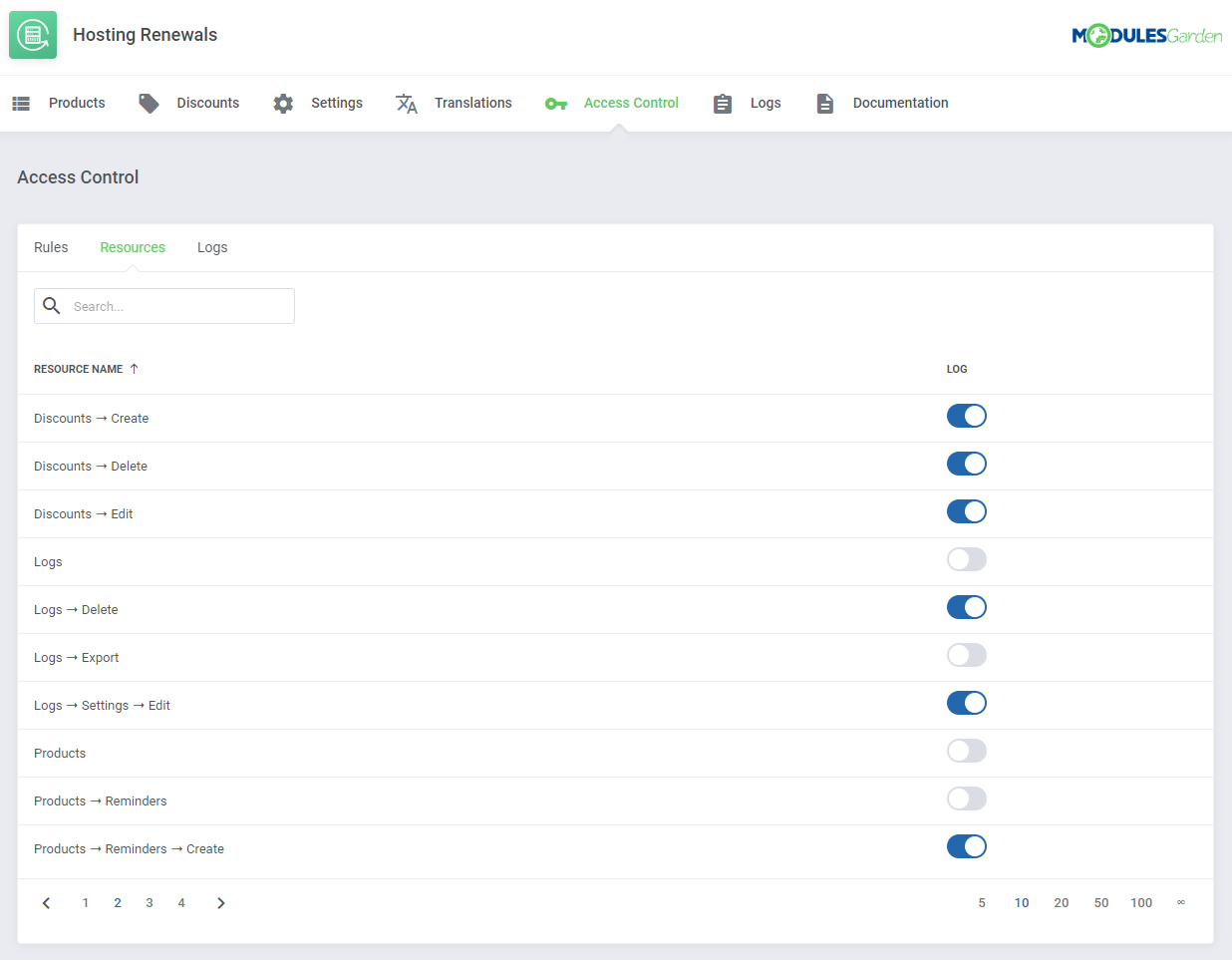In this detailed screenshot, we see the user interface of an application or website titled "Modules Garden." The title "Hosting Renewals" is prominently displayed in the upper left corner, indicating the section of the application currently being viewed. On the upper right corner, the branding "Modules Garden" is highlighted in blue and green, further identifying the application.

The interface includes a navigational panel with several sections such as Products, Discounts, Settings, Translations, Access Control, Logs, and Documentation. The "Access Control" section is currently active, indicated by a green highlight.

Within the "Access Control" section, there are subsections labeled Rules, Resources, and Logs. The view is currently focused on the "Resources" subsection, which features a search box and a table listing various resources. Each resource entry includes different permissions like create, delete, edit for sections such as Discounts, Logs, and Products. For instance, there are controls for Discounts (Create, Delete, Edit), Logs (Delete, Export, Settings Edit), and Products (Reminders Create).

Towards the bottom of the screen, pagination options indicate that there are four pages available for navigation, along with a dropdown menu to modify the number of entries displayed per page, ranging from 10 to 100 entries. Currently, 10 entries are being displayed per page, suggesting the existence of approximately 40 different permission toggles, some active and some inactive. Overall, the screenshot provides a comprehensive view of the access control management within the Modules Garden application.